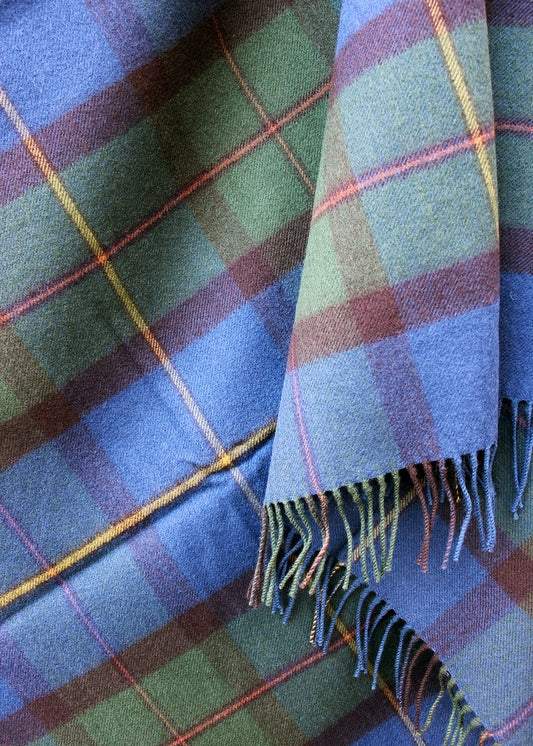This image depicts a vibrant plaid flannel fabric, possibly a blanket or tablecloth, folded and draped to showcase its intricate design and frayed edges. The vertical photograph captures a rectangular piece of fabric featuring a checkered pattern with alternating blue and green squares, intersected by bold half-inch red lines. These red lines, when layered over the squares, create subtle shifts in color, rendering purplish hues over the blue squares and orange tones over the green ones. Complementing this colorful palette are thin yellow lines that traverse both horizontally and vertically across the fabric, adding a lively contrast.

On close inspection, the red lines appear almost pink due to their brightness, adding another layer of visual interest. The fabric displays signs of wear with strings hanging from the edges, introducing a sense of texture and depth to the image. The top left corner of the image features a portion of fabric meticulously folded over, mirroring the vibrant criteria of the rest of the fabric—blue, green, blue panels segmented by yellow and red lines.

Overall, the vivid patchwork captured in the photograph combines hues of blue, green, yellow, and red, creating an eye-catching composition that's both aesthetically pleasing and practically versatile, ideal as a cozy sofa throw or decorative bedspread.